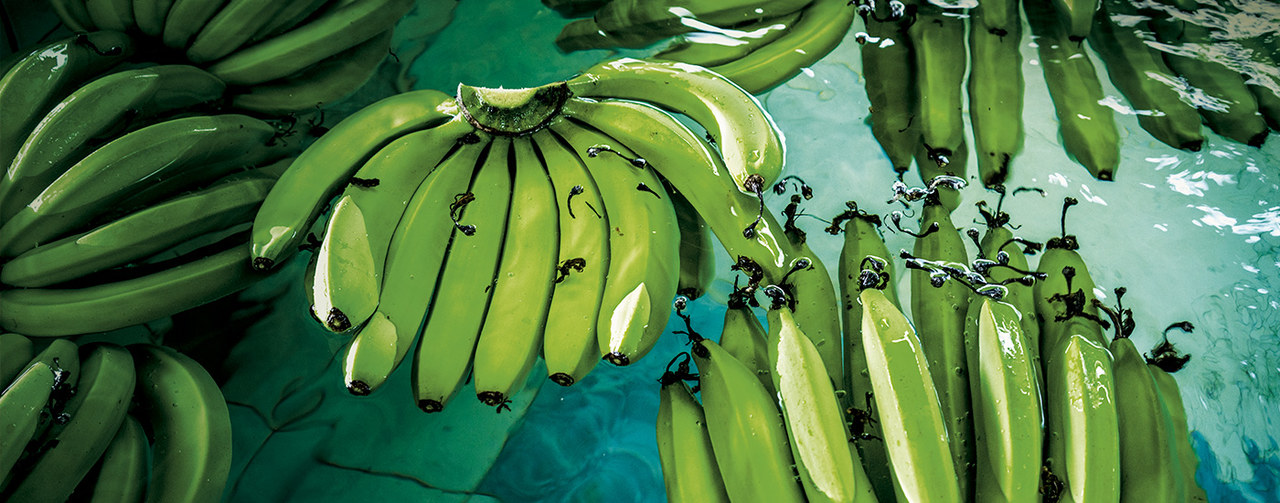The image is a rectangular panoramic photograph featuring a surreal scene of several large bunches of green, unripe bananas floating in clear blue water. The scene appears to be either a swimming pool or an ocean, with clean blue water suggesting the former. On the left side of the image, the edge of the water is visible with some rocks nearby. Scattered through the water are six and a half visible banana bunches, each containing approximately 15 bananas. Some of these bunches are facing curved side up, revealing the cut stems. The bottom right of the image shows what could be aquatic plants. Notably, the bananas display black curly stem ends, which resemble insect-like structures. The left side of the image is densely filled with these green banana bunches, making for a visually arresting and unusual composition.